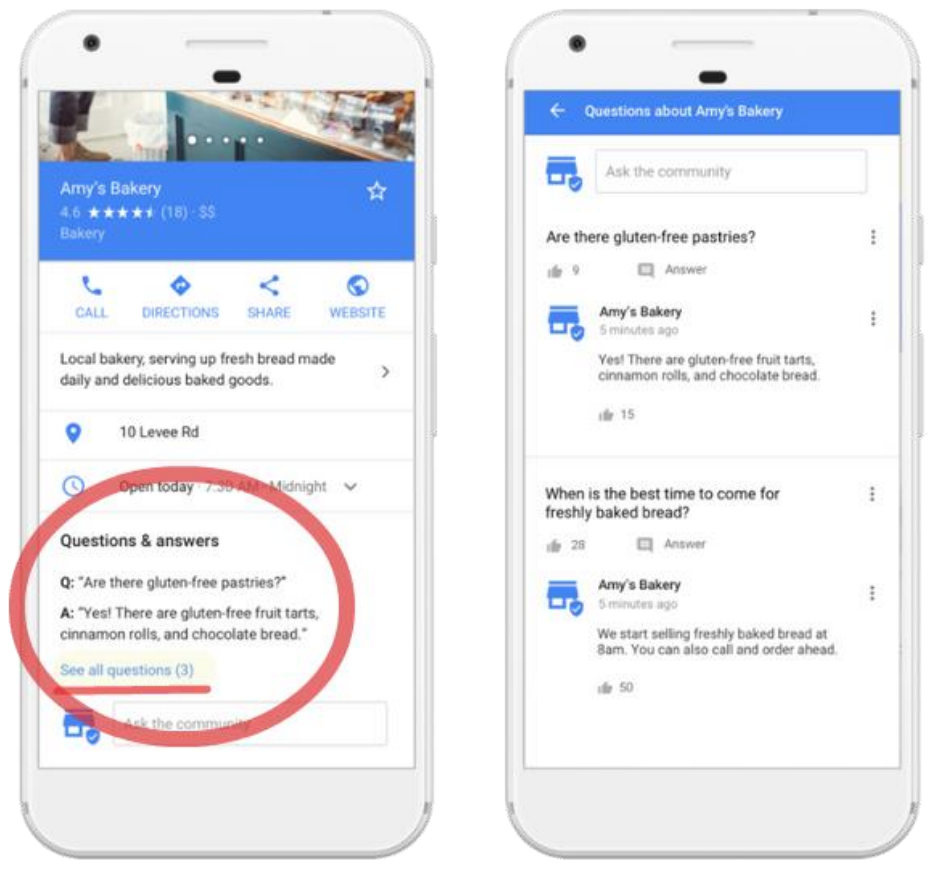This detailed image showcases a screenshot of two AI-generated smartphones, both with a realistic superimposed screen display. The phones, rectangular with rounded edges and whitish in color, are positioned side-by-side in portrait orientation.

On the left phone, the screen's top displays a blue header bearing the text "Amy's Bakery" in white. It features a 4.6 star rating based on 18 reviews, indicates a moderate price range with two dollar signs, and includes a hollow star icon for favoriting. Below this, "Bakery" is labeled explicitly. The screen displays thumbnail images of the bakery with navigation dots to scroll, although this section is partially cropped.

Further down, under a white background, a row of blue icons for calling, getting directions, sharing, and viewing the website is visible. Below, a gray line separates the icons from a brief description, stating, "Local bakery serving fresh bread made daily and delicious baked goods." Another bordered section follows, beginning with a blue pinpoint icon for the address and a blue clock icon indicating hours of operation. 

Prominently, there's a red circle emphasizing a section titled "Questions & Answers." Here, a user inquires, "Are these gluten-free pastries?" The bakery confirms: "Yes, they are gluten-free fruit tarts, cinnamon rolls, and chocolate bread."

On the right phone, the screen is titled "Questions about Amy's Bakery" in a blue box with white text. It restates the gluten-free pastries query, providing the same response from Amy's Bakery. Additionally, another question asks, "When is the best time to come for freshly baked bread?" The bakery's reply suggests that bread is available starting at 8 a.m., with an option to call and order in advance. Essentially, this phone reiterates the same information as the left, but in an alternate format for user convenience.